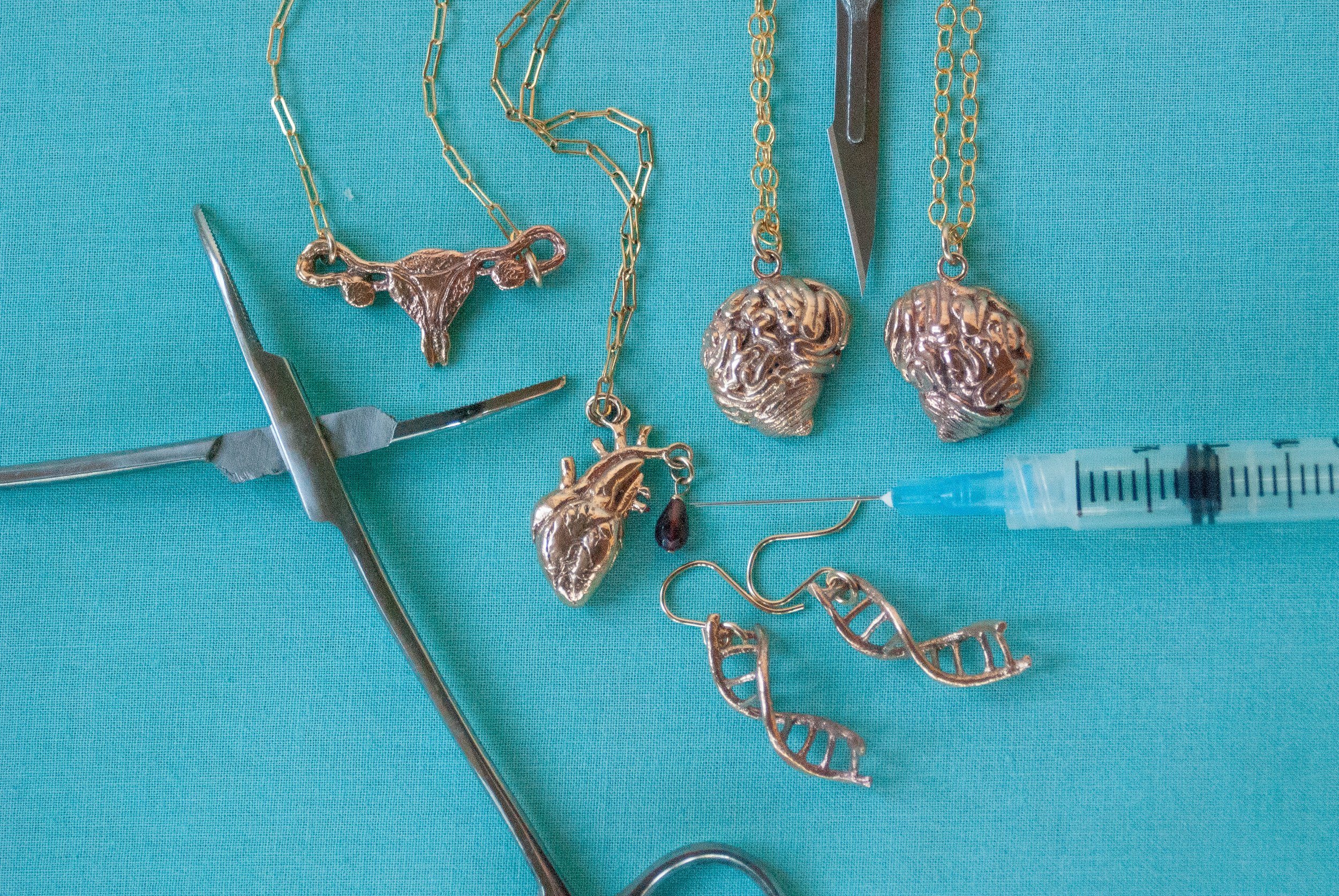The image depicts a collection of assorted objects laid out on a blue fabric surface, possibly resembling medical or hospital tray covers. Key elements include a pair of open silver scissors, likely for clipping nails, and a sharp metal dagger positioned somewhat off-frame. Adjacent to these is a clear syringe with black markings and a blue cap, with the needle itself silver. The scene also showcases various pieces of coppery gold jewelry with square-loop chains. One chain holds a pendant in the shape of a bull's or cow's head, another a heart with an attached black bead. Two other chains feature pendants resembling brains. Additionally, there are a set of coppery gold earrings shaped like twisted ladders or DNA helices. All items are meticulously arranged without any accompanying text.